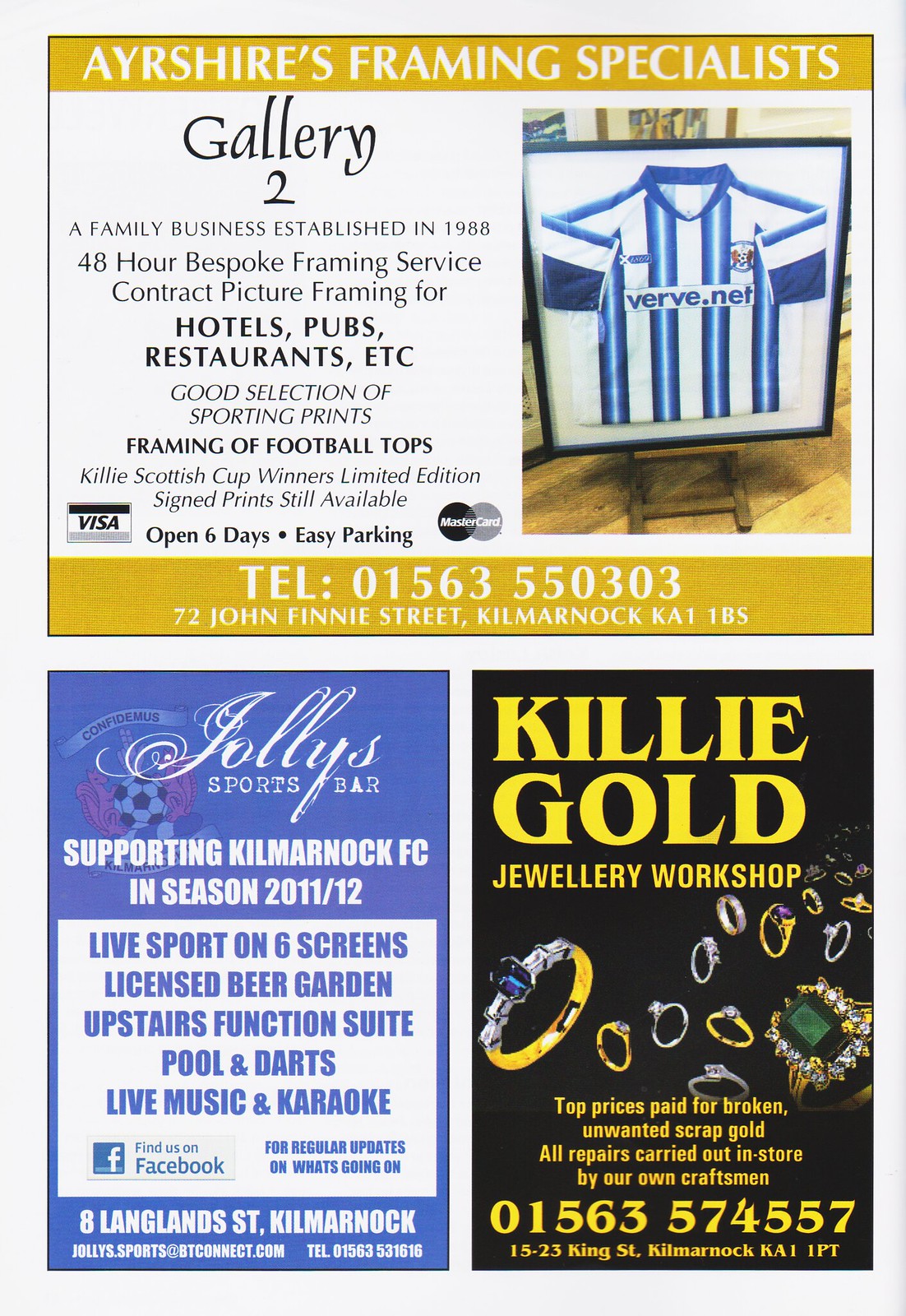The image features a comprehensive advertisement page likely from a magazine or flyer showcasing three distinct businesses. At the top, on a yellow stripe with white text, it reads "Ayrshire's Framing Specialist," emphasizing a family business known as Gallery, established in 1988. The advertisement highlights a 48-hour bespoke framing service and offers picture framing for hotels, pubs, and restaurants, alongside a selection of sporting prints and football tops. Featured prominently is a framed soccer jersey in a white frame, and a special mention of a Killey Scottish Cup Winners Limited Edition signed print still available. Payment options include Visa and MasterCard, and the business is open six days a week with easy parking.

Below this ad, on the left, is an advertisement for Jolley Sports Bar, supporting Kilmarnock FC in the 2011-12 season. The ad, predominantly blue, details live sports on six screens, a licensed beer garden, an upstairs function suite, pool and darts, and live music and karaoke.

To the right, a black and yellow ad for Killey Gold Jewelry Shop showcases flying silver and gold rings. It mentions top prices paid for broken, unwanted, and scrap gold, with all repairs conducted in-store by their own craftsmen. This section also provides a contact number and address.